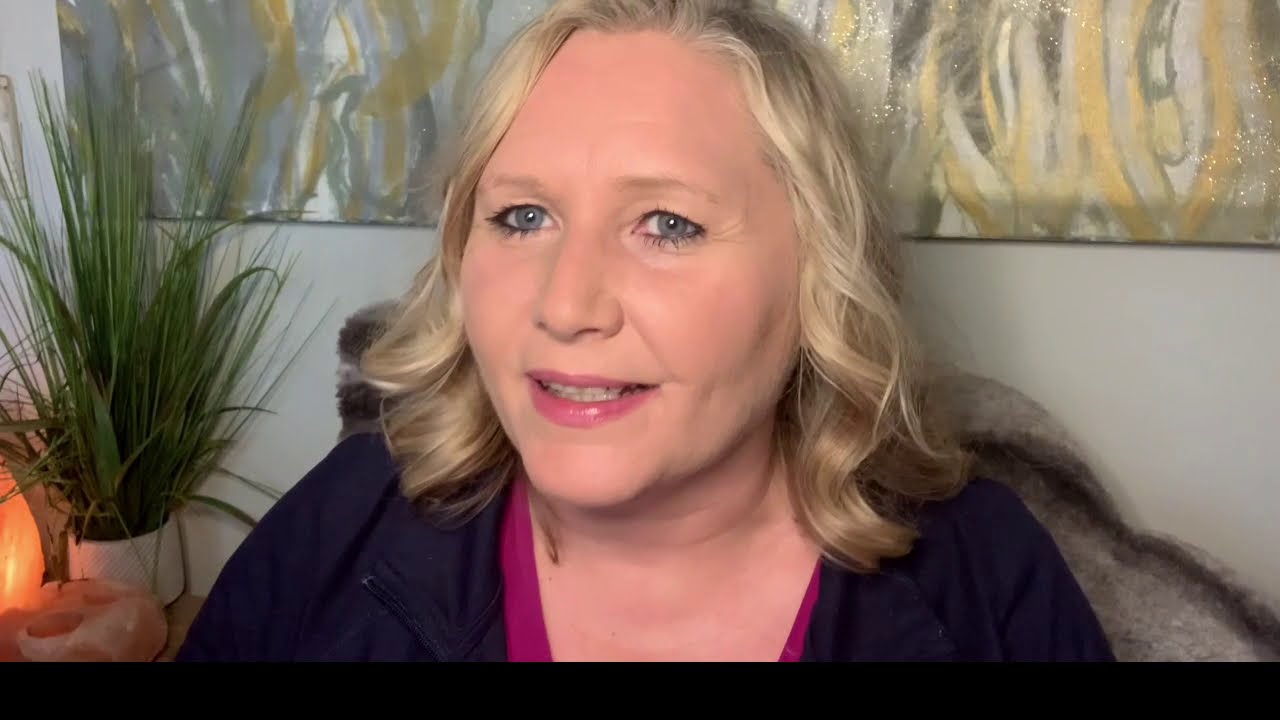This high-definition image captures a close-up of a Caucasian woman appearing to be in her 40s, who is speaking, perhaps indicative of a video frame. She has shoulder-length, curled blonde hair framing her round, wide face, adorned with pink lipstick and mascara, and bright blue eyes. She is dressed in a dark blue jacket over a pink v-neck blouse and is smiling gently with her mouth open, revealing both her top and bottom teeth. The scene is set in what seems to be a cozy, possibly holistic office or home environment, with beige walls casting a slight greenish hue. Behind her, there is an abstract, modern painting featuring vertical squiggly lines in shades of yellow, gray, and white with gold speckles. To her right, a small end table holds a white potted plant with tall, green stalks—some curling at the ends—and a pink salt lamp, adding a touch of tranquility to the setting.